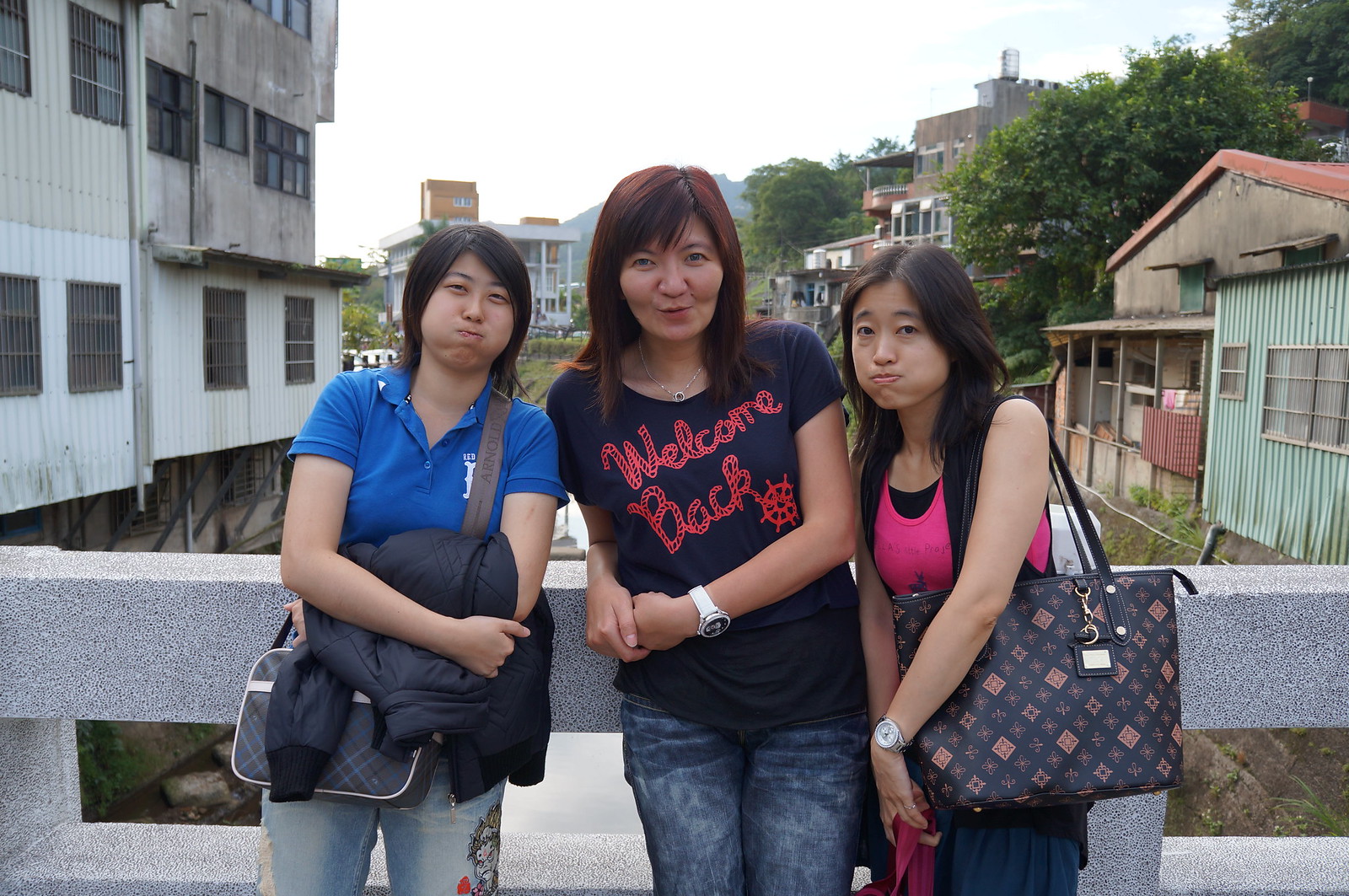The photograph features three Asian women standing on a bridge that connects two apartment buildings in a small neighborhood town. The woman on the left is wearing a blue polo short-sleeved shirt with a collar and a design on the left chest area. She is holding a blue jacket folded around her forearm. The woman in the middle, who is notably taller, is dressed in a black t-shirt that says "Welcome Back" in stylized red text and blue denim pants. The woman on the right wears a pink tank top over a black t-shirt and carries a large black designer bag. Each woman is making a playful pouty face by blowing out their cheeks, giving the impression that their mouths are full or that they are holding their breath, adding a humorous touch to the scene. All three appear to be smiling and laughing, suggesting an inside joke or shared funny moment. Behind them, the neighborhood town with old, somewhat unmaintained buildings and abundant trees is visible, providing a backdrop to this candid and lighthearted moment.